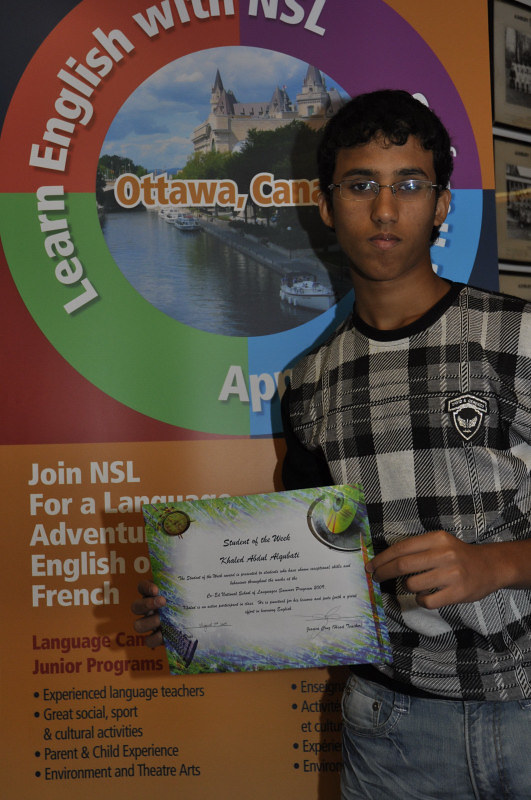A young boy, approximately 12 or 13 years old with medium skin tone and black hair, is holding up a certificate in front of a large, colorful poster. The poster features a prominent circle at the top with vibrant hues of red, purple, blue, and green, and white text that says "Learn English with NSL." In the center of the circle, it reads "Ottawa, Canada" and includes an image that appears to depict the Parliament building or a canal scene from Ottawa. Below this, the poster has an orange background with text that reads "Join NSL for a language adventure" and details about the program, including "experienced language teachers," "great social, sport, and other cultural activities," among other descriptions, which are partially obscured by the boy holding the certificate.

The boy, identified by the certificate as Khaled Abdul-Ajoubadi, student of the week, is wearing black-rimmed glasses, a black, gray, and white flannel-looking shirt with a crest patch on the right chest area, and blue jeans. He's positioned slightly to his right, proudly displaying his achievement. He's in an English learning environment, possibly part of a junior language program. The certificate features a green and blue design along its edges, though the smaller text on it is not clearly readable.